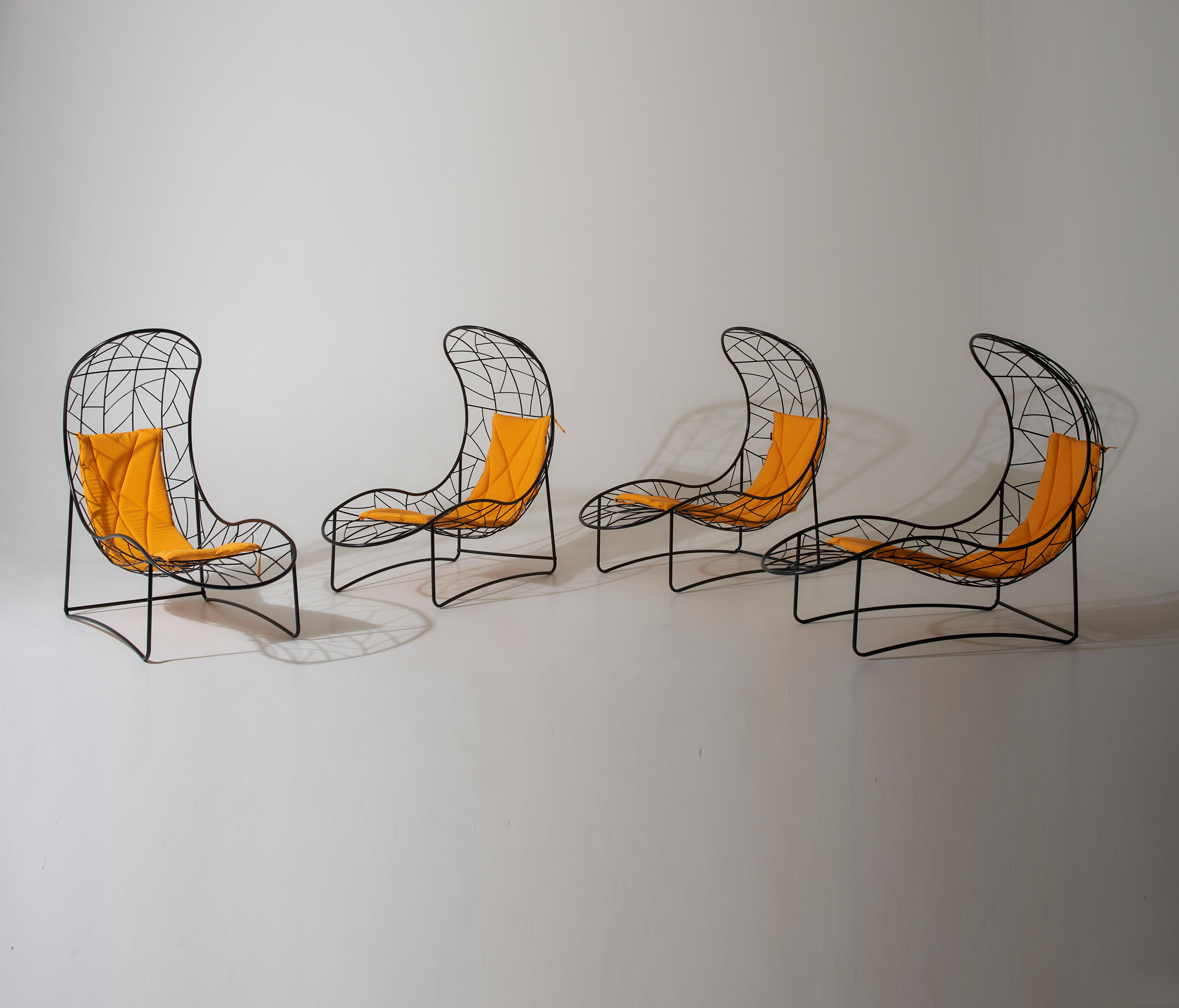This image showcases a set of four minimalist curved wire chairs arranged in a semi-circle against a grayish white background. The chairs are constructed from black metal, featuring a dramatic open and airy design with a see-through woven pattern. They possess a swooping backrest that extends from the seat, resembling a curled shape akin to a potato chip, with a connecting rod between the two legs at the back. Each chair is adorned with a thin, yet foamy orange cushion that provides the only color contrast in this otherwise monochromatic scene. Despite their modern and possibly outdoor aesthetic, the chairs do not seem to be part of any home or patio setting, emphasizing the simplicity of the composition. The cushions are designed to follow the ergonomic curve of the chairs, supporting from the neck down to the knees. This setup suggests that the chairs offer a lounging experience, although they may not fully elevate the legs.